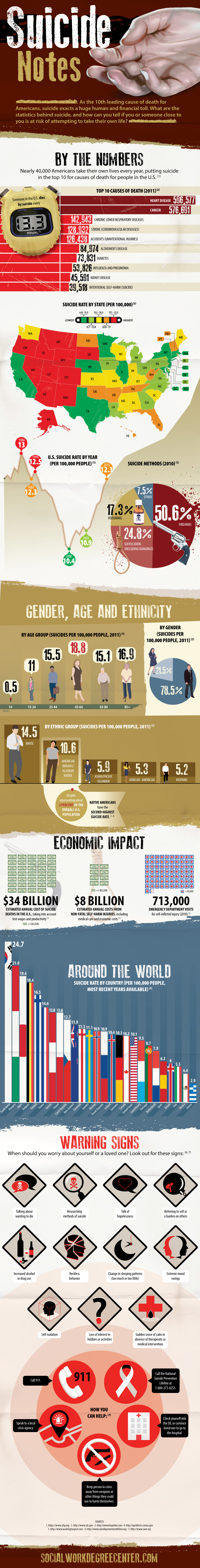The poster is long and rectangular.

At the top, there is a brown rectangular section with the word "Suicide" written in white in the upper left-hand corner. Beneath this, in light brown, it says "Notes". To the right of the text, an illustration of a feather, colored pale rose, white, and gray, is present.

Below this header, a large beige square is divided. The upper half features a white background with a colored map of the United States, marked in red, green, yellow, and orange. There is text above and below the map.

The section beneath the map comprises a tan rectangle with symbols, numbers, and white text. Following that, there is a white strip with the text "Economic Impact" centered in black. Under this strip, there are three separate images set side-by-side, each accompanied by dollar figures.

Lower down, a slate blue rectangle gives the appearance of books lined up on a shelf, but on closer inspection, they are flags of countries. Centered at the top of this section in white text, it reads "Around the World". Below this, a white square contains sideways diamonds with symbols inside.

At the very bottom of the poster, there is a thin strip of brown.